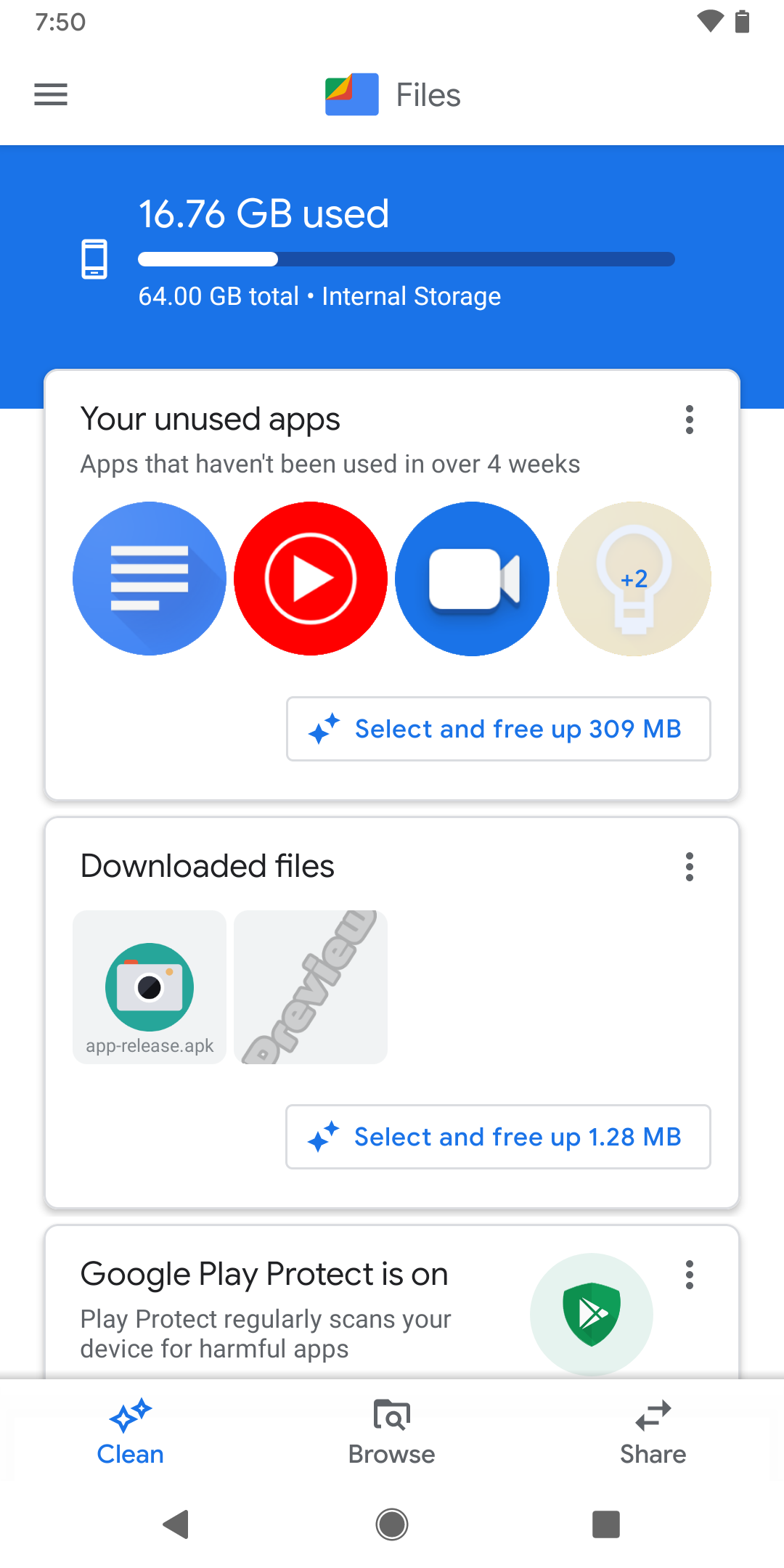The image depicts a vertically-oriented screenshot, likely taken from an Android or iPhone. The screenshot captures a device’s storage management interface with a predominantly white background containing various icons, figures, and text.

At the very top of the image, there are typical status bar indicators:
- In the upper left corner, the time is displayed as "7:50" in black text.
- On the far right of the same row, there is a black Wi-Fi symbol and a fully charged black battery icon.
- Below the time, three horizontal lines are stacked, resembling a menu icon.
- Centered on the same row is a blue square with a torn upper left corner revealing green, yellow, and red pages underneath. Below this icon, the word "Files" is displayed in black text.

The central portion of the screenshot features a sizeable blue rectangle slightly offset to the left with the text "16.76 GB used" written in white letters. Immediately beneath it, a line approximately one-third filled with white transitions to a dark blue background. The line represents internal storage capacity, with "64.00 GB total" indicated below it in white text. Adjacent to the line on the left is an icon of a mobile phone.

Further down, a white box partially overlaps the blue rectangle. The upper left of this box reads "Your unused apps" in bold black text, with a subheader stating "Apps that haven't been used in over four weeks" colored in black as well. In the upper right corner, three vertical dots signify a menu option.

Below this, four circular icons are visible:
1. A blue circle with three long vertical lines and one shorter white line in the middle.
2. A red circle featuring a white play button.
3. A blue circle with a white video camera icon.
4. A dimmed icon similar to the red one but featuring a blue plus sign.

Towards the lower right corner of this box, there's a gray-rimmed box with two blue stars and adjacent text in blue reading "Select and free up 309 MB."

Lower down, another gray-rimmed white box appears with the top left text stating "Download 5 downloaded files" in black. This section features:
- A gray square with a teal circle centered with a gray camera icon.
- A second gray square displaying "Preview" in gray lettering angled from the lower left to the upper right.
- Further down, three stacked dots appear on the upper right of another gray-rimmed rectangle, which contains blue stars to the left and further right reads "Select and free 1.28 MB" in blue text.

Finally, the image cuts off, revealing part of the section labeled "Google Play Protect is on" with underlying gray text indicating "Play Protect regularly scans your device for harmful apps." Adjacent to this is a pale green circle with a green shield and white shield images inside it, with three vertical dots in the upper right corner.

In the lower part of the white area, two blue stars are labeled "Clean" in blue, a folder with a black magnifying glass icon, the word "Browsing" in black text, left and right-facing arrows, and the text "Share" in black. At the very bottom, there is a black play button icon and a small black square on the far right.

Overall, the image meticulously details the storage management and app usage insights of the device’s interface, providing a clear view of the system's status and potential actions for optimization.